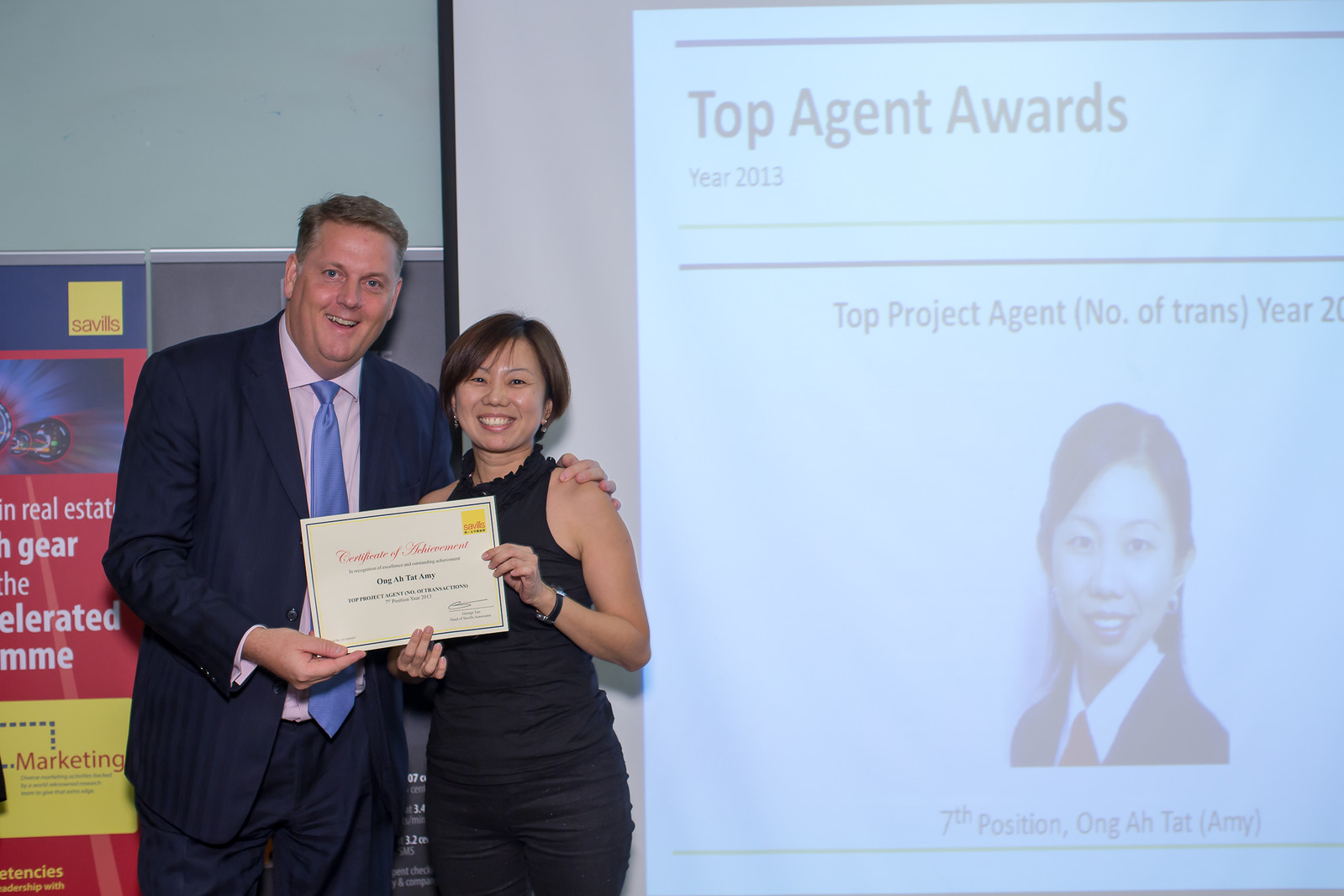This photograph captures a jubilant moment between two individuals during an award ceremony. On the left stands a white man, appearing in his late 40s to 50s, with graying brown hair. He is dressed in a dark blue pinstriped suit, complemented by a light blue tie and a white button-down shirt. Beside him, to the right, is an Asian woman in her 40s, with short black hair. She is elegantly dressed in a black sleeveless dress and black pants. 

Both are smiling warmly at the camera while holding a certificate of achievement between them. The man seems to be presenting the award to the woman. Behind them, a projector screen displays a slide that reads "Top Agent Awards, Year 2013, Top Project Agent," although part of the text is cut off. Below the text is a headshot of the woman and the words "7th Position, Ong Ah Tat (Amy)." The moment signifies recognition and celebration of the woman's accomplishments, as they jointly display the award for the photograph.